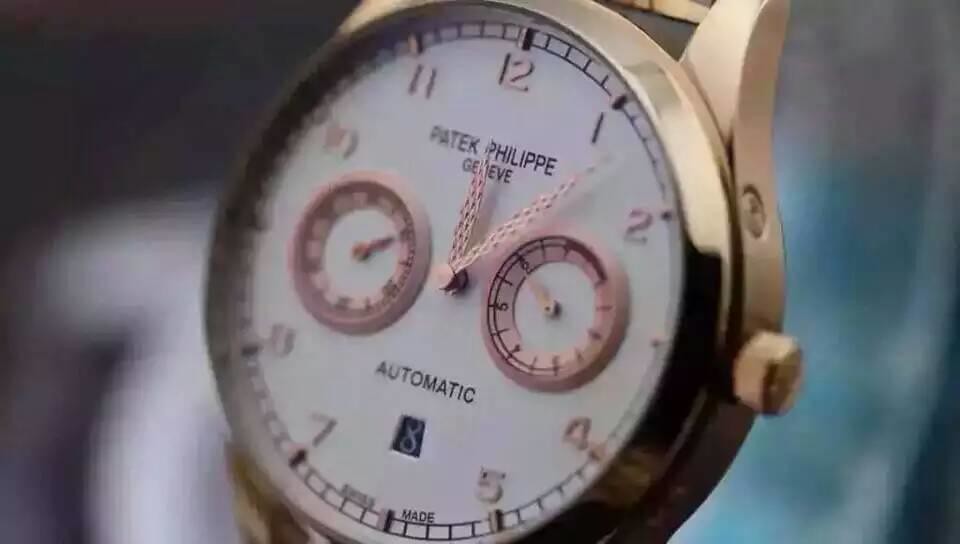This is an extremely close-up photograph of a Patek Philippe watch face, showcasing its exquisite details against a blurred, predominantly blue and white background. The watch housing appears to be made of gold or highly polished brass. The dial is white with black text, prominently displaying "Patek Philippe" at the top and "Genève" underneath. The face features numerals in a standard format as opposed to Roman numerals, with additional markers for precision. The watch shows the time as five minutes past twelve, indicated by two elegant rose gold or copper-colored hands. There are two small sub-dials side-by-side, crafted from the same rose-gold material, presumably detailing seconds and possibly another function. A slight cutout reveals a date, showing the number 8 on a black background. The overall composition emphasizes the luxurious and intricate design of this vintage-looking, high-end watch.